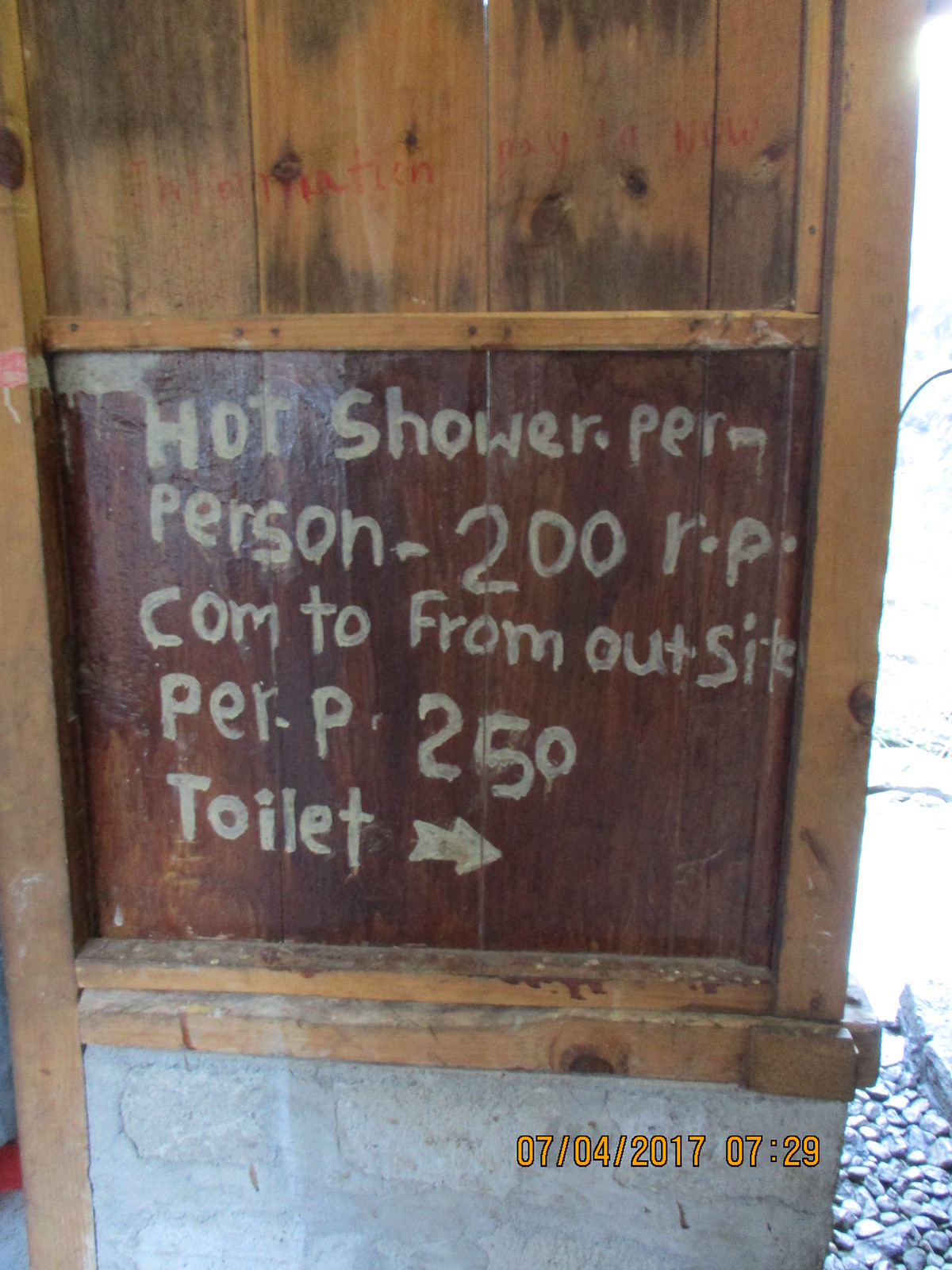The photograph captures a weathered, wooden wall with a homemade sign crudely painted in white and yellowish paint. The sign reads, in uneven letters, "Hot shower per person 200 RP. Come to from outside per P 250. Toilet," with an arrow pointing in the direction of the toilet. The wooden structure appears aged and rustic, contributing to a sense of an outdoor, daytime setting. In the lower portion of the image, digital text indicates the date and time: July 4th, 2017, at 7:29. The entire image is vertically oriented with the painted letters centered and the digital timestamp positioned towards the bottom right corner. Hues of brown, beige, tan, gray, white, and yellow dominate the color palette.